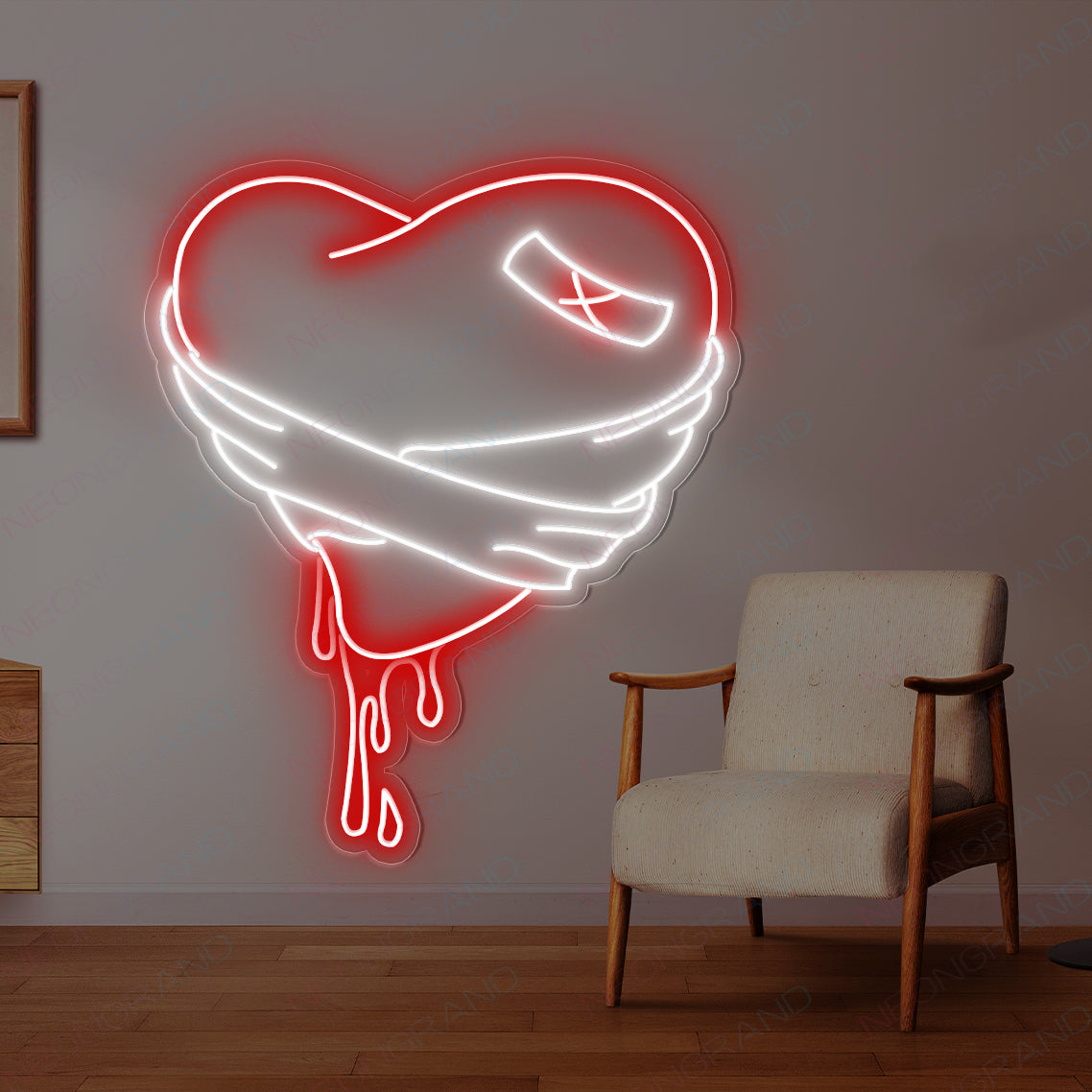This photograph captures a dimly lit room with a striking, large neon sign on the wall. The neon sign, glowing in vibrant red, is shaped like a heart with evocative blood drips cascading from it. The heart is wrapped with white bandages forming an X shape, and a white bandage is also visible on one corner, rendered in neon lights. The heart sign, framed by a subtle outline, is positioned in the top left quadrant of the image, casting an intense, bright glow that contrasts starkly with the dimly lit grey walls and the light brown hardwood floor. Below the sign, towards the right, is a small white chair, its light grey fabric upholstery accented by medium brown wooden arms and legs. The chair is slightly angled towards the viewer, adding depth to the scene. In the left corner of the image, partially visible, is a wooden dresser with a mirror mounted above it, further enriching the room's aesthetic. The overall ambiance of the photograph is moody and focused, emphasizing the glowing heart as the visual centerpiece.